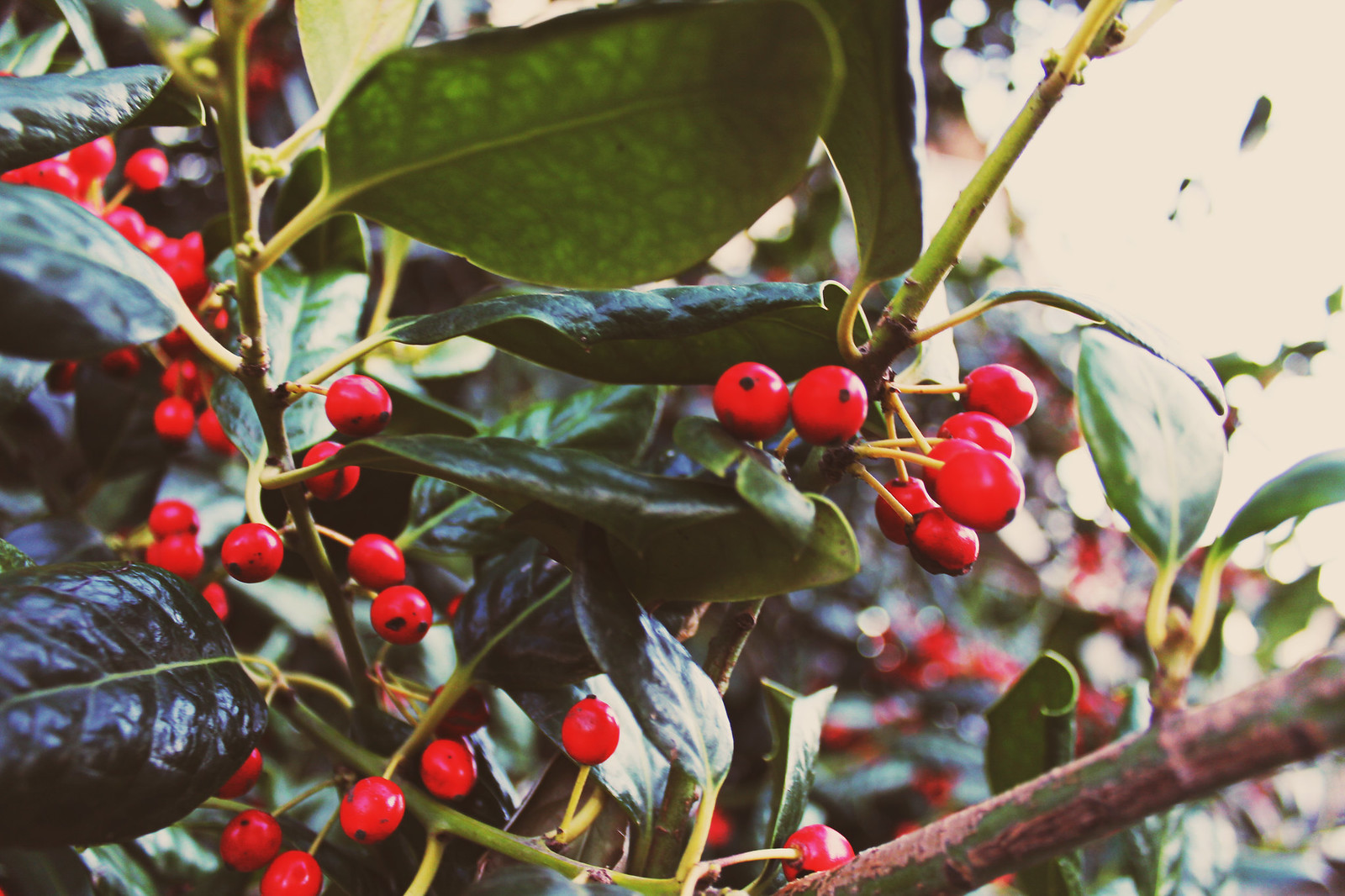This image portrays a natural scene featuring a coffee plant outdoors during the daytime. The composition is dominated by clusters of bright red berries resembling coffee beans, each perched on small yellow stems and marked with a distinctive black dot at their tips. These berries are nestled amongst a variety of leaves, ranging from dark, almost forest green with a rich texture to newer, lighter green shoots sprouting from the thicker branches. Notable is a robust, partially green branch with a touch of pinkish hues, hinting at the plant's vigorous growth. Sunlight filters softly from the upper right corner, highlighting the plant's details, casting a gentle illumination across the scene, and enhancing the natural vibrancy of the leaves and berries, creating a serene and well-lit outdoor atmosphere.